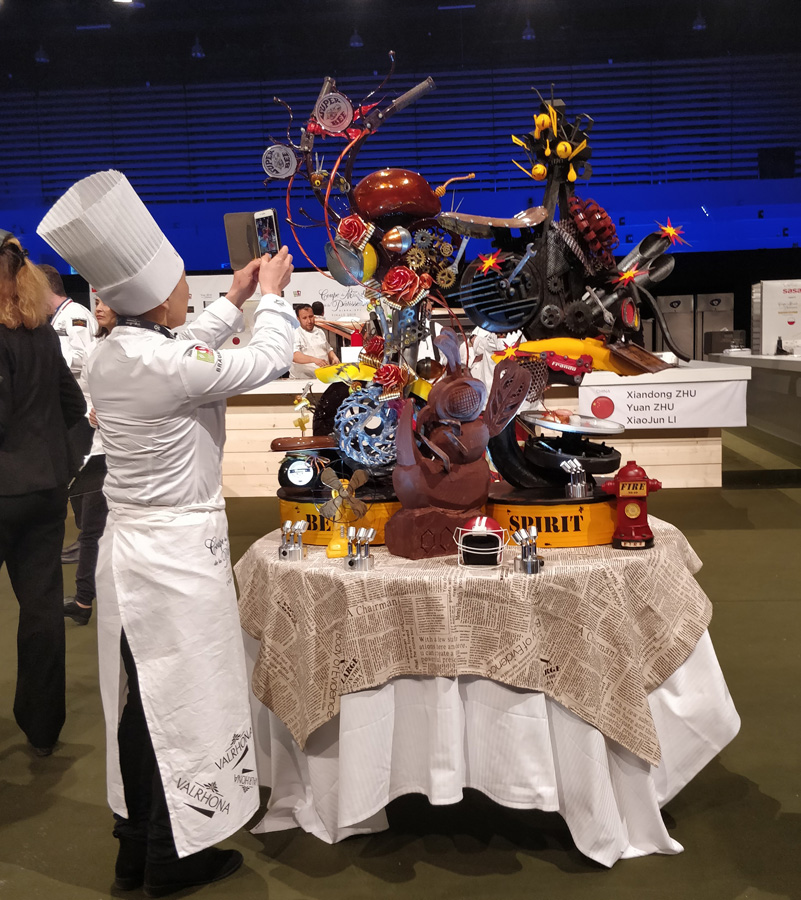This photograph captures a chocolate dessert competition held in an indoor space with a white and newspaper-print tablecloth-draped round table at its center. The main focus of the image is a complex, metal-like structure resembling a motorcycle, incorporating a yellow platform with the word "Spirit" on it. The creation includes various components such as handlebars, a bicycle-like seat, wrenches, tailpipes, and wheels, all artistically constructed from chocolate and spun sugar and painted to mimic real motorcycle parts. Nestled among these elements are additional items like a miniature fire hydrant labeled "Fire," a small fan, little lights, and a football helmet.

In the foreground, a female chef with her back turned to the camera is capturing the intricate chocolate sculpture with a smartphone. She is dressed in a tall chef's hat, a white long-sleeved shirt, a white apron, and black pants. The background reveals more individuals in white chef jackets and black pants, emphasizing the culinary theme of the event. A man is visible standing at a counter with a sign above him containing multiple lines of text written in what appears to be Chinese characters.

The room is lit with fluorescent lighting, highlighting the taupe-brown floor and white and blue-lit back wall. Overall, the detailed and creative centerpiece stands out as a remarkable piece of edible artistry within the bustling, culinary environment.